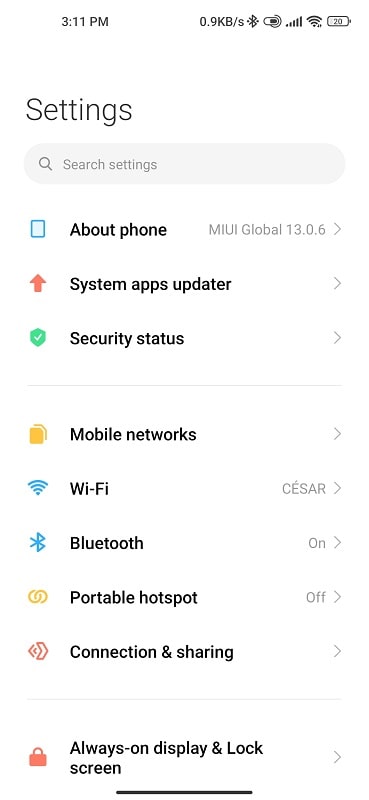The image depicts a detailed view of a cell phone's settings page, set against a plain white background. At the top of the screen, the time is displayed as 3:11 PM, with additional indicators to the right showing the phone's signal strength, battery life, and other status icons. 

The settings page begins with a search bar labeled "Search settings." Below this, a series of menu items are listed: "About the phone," "System apps updater," and "Security status." Each of these options is accompanied by distinct small icons: "About the phone" has a blue square, "System apps updater" features a red arrow, and "Security status" displays a green shield.

A thin gray line separates the initial section from the next set of options, which includes "Mobile networks," "Wi-Fi," "Bluetooth," "Portable hotspot," and "Connection and sharing," all of which are denoted with corresponding icons, such as the recognizable blue Wi-Fi symbol.

Another thin gray line demarcates the aforementioned options from additional settings, labeled "Always on display and lock screen." Each item on the list is written in black text, making it easy to read against the white background.

Overall, the image provides a comprehensive and organized look at the various settings available on a cell phone, with clear visual cues to aid in navigation.